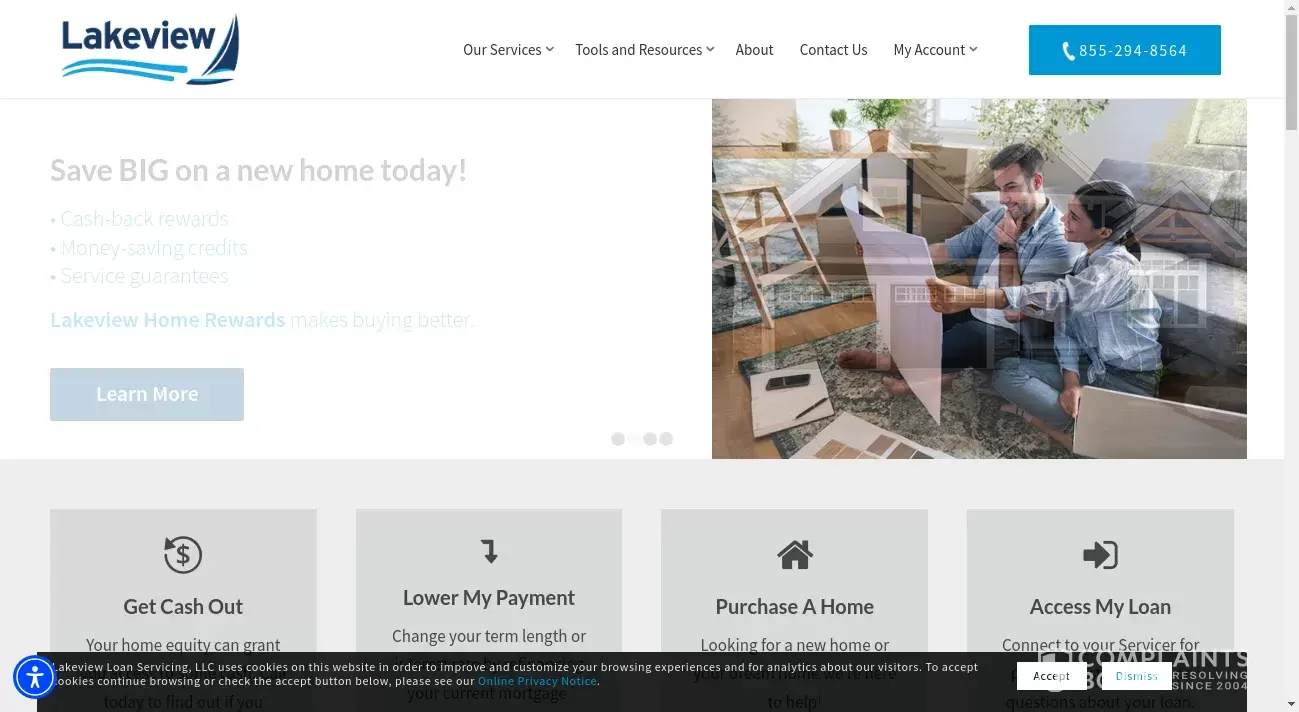In the image, a web page with a white background is displayed. At the top, the title "Lake View" is showcased in blue font accompanied by a sailboat graphic and two wave motifs representing water. The navigation bar at the top includes options: "Our Services" with a downward arrow, "Tools and Resources" with an arrow down, "About," "Contact Us," and "My Account" with an arrow down.

Below the navigation bar is a blue strip featuring white text and a phone handset icon, displaying the number 855-294-8564. The main banner headline reads, "Turn Home Equity into Cash, Jumpstart Your Plans and Achieve Your Dreams," followed by a prominent blue button labeled "Get Started."

The central part of the page showcases a photograph of a man and a woman sitting on the floor in a cozy living room area against a gray couch. Both are smiling and holding a large piece of white paper, seemingly engaged in planning home improvement projects. Various swatches are scattered on the ground around them, along with a pen, a tablet, and a mobile phone, all placed on a small area rug.

At the bottom of the image, there is a gray button with multiple options: "Get Cash Out," "Lower My Payment," "Purchase a Home," and "Access My Loan."